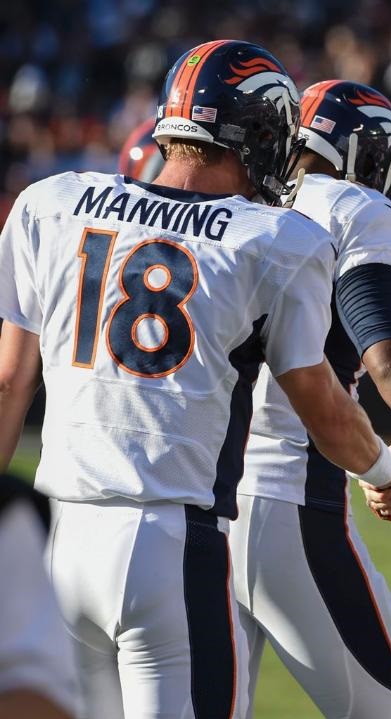The photograph captures two Denver Broncos football players from behind, prominently featuring a player identified by his white jersey with blue trim that reads "Manning, 18," with the "18" outlined in orange. The player, likely Peyton Manning, stands wearing a distinctive blue and orange helmet adorned with the Broncos emblem—a white horse with orange mane—on the side, and an orange stripe down the center. His jersey and matching white pants feature a dark blue stripe with a touch of orange trim running from under his arm to the side of his leg. In front of Manning, another player in an identical uniform partially obstructs the view, making their name and number indiscernible. The background reveals a blurred crowd, possibly spectators, and a grassy field, indicating an in-game moment at a football match.